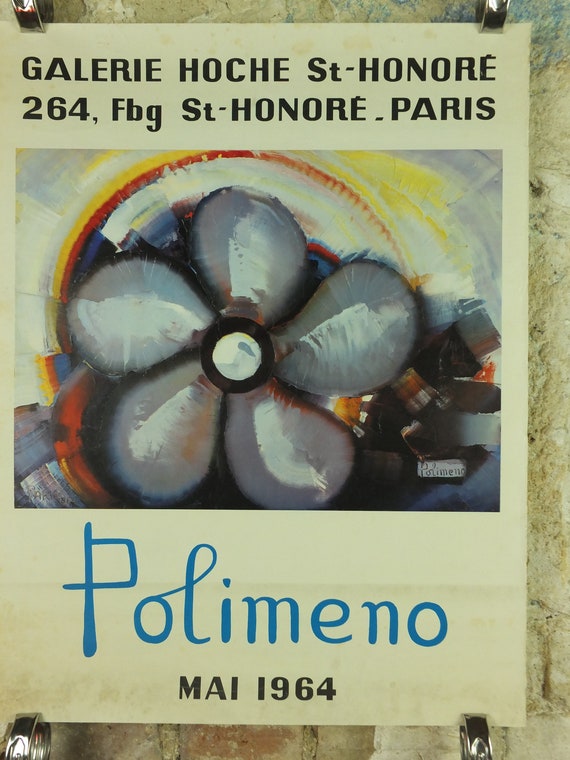This vintage advertisement flyer, pinned to a wall, announces an event at Gallery Hoche Saint-Honoré, located at 264 FBG Saint-Honoré, Paris. The focal point of the flyer is an abstract illustration in the center, which resembles either a flower or a boat motor's fan blades, featuring five solid white blades in motion. The movement is vividly depicted with yellow and red hues creating a dynamic effect. The flyer displays aging around its edges, enhancing its nostalgic feel. Below the illustration, in prominent blue text, is the name "Palomino," followed by "May 1964" in smaller black text, indicating the event date.